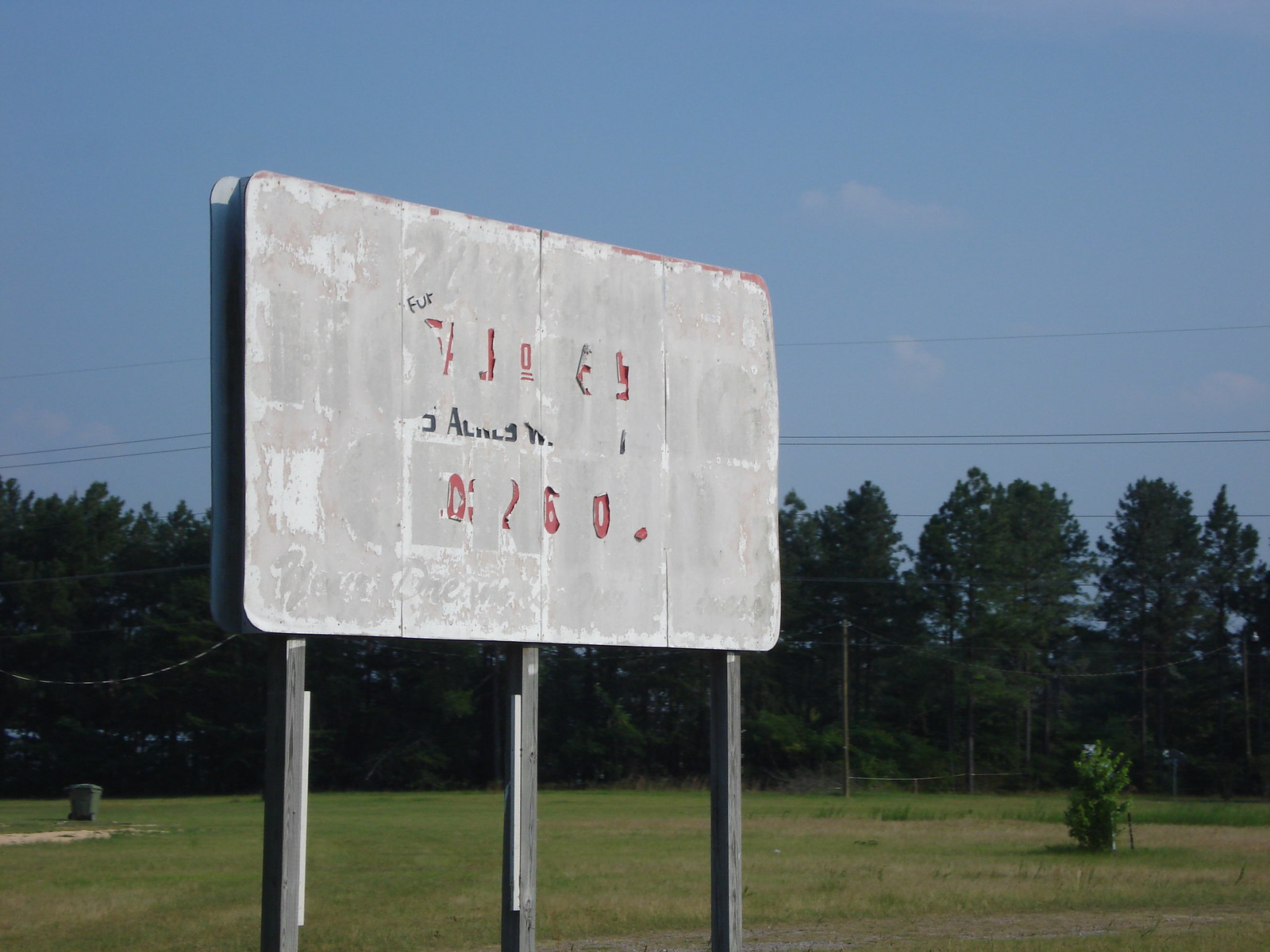In a desolate and rundown country area stands an aged and weathered billboard. Its once vivid colors have faded, leaving a predominantly white surface with remnants of red and black lettering. The most legible part of the advertisement is the number "260." The word "fur" is faintly visible in the upper corner, though it's unclear whether it's the right or left side. The billboard is supported by three old, faded wooden beams, adding to its dilapidated charm.

In the surrounding landscape, a gray trash can is situated to the left, while a small tree or large shrub grows on the right. The backdrop features a meadow, with a neatly lined row of mature trees framing the scene.